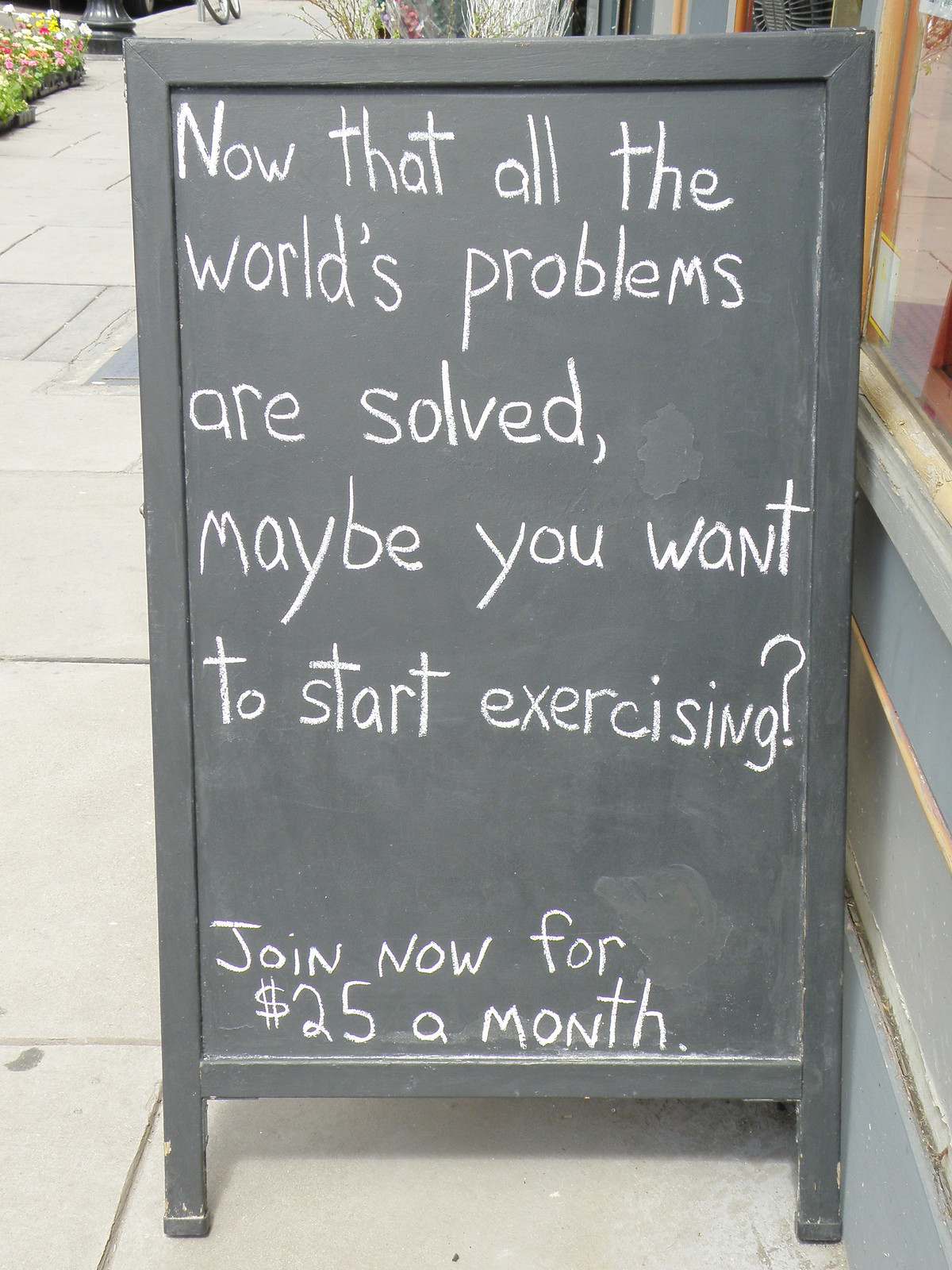This photograph displays an outdoor chalkboard sign positioned on a paved walkway in front of a gym building. The sign, resembling a sandwich board or A-frame commonly found outside restaurants, sits against the gray wall of the building, with part of a window visible on the right side. The sign is black with white, somewhat messy handwriting in chalk. It reads, "Now that all the world's problems are solved, maybe you want to start exercising? Join now for $25 a month." On the left side of the image, there's a sidewalk where colorful flowers and planters can be seen, suggesting an urban setting with some greenery.